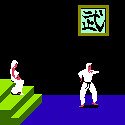This image, roughly 1 inch by 1 inch, appears to be a pixelated screenshot from an early 90s video game. The background is predominantly black, with a royal blue floor at the bottom. On the left-hand side, there are three lime green steps descending towards the blue floor. On the middle step stands a female figure dressed in a white outfit with a hood or head covering, while a man in a white martial arts outfit with a black belt stands at the base of the steps. He seems to be engaged in an activity reminiscent of tai chi, judo, or another martial art. Both characters have brown or reddish shoes. Above the man, in the top right corner of the image, there is a small square painting with a brown frame and a light blue center, adorned with what appears to be black Chinese or Japanese characters.